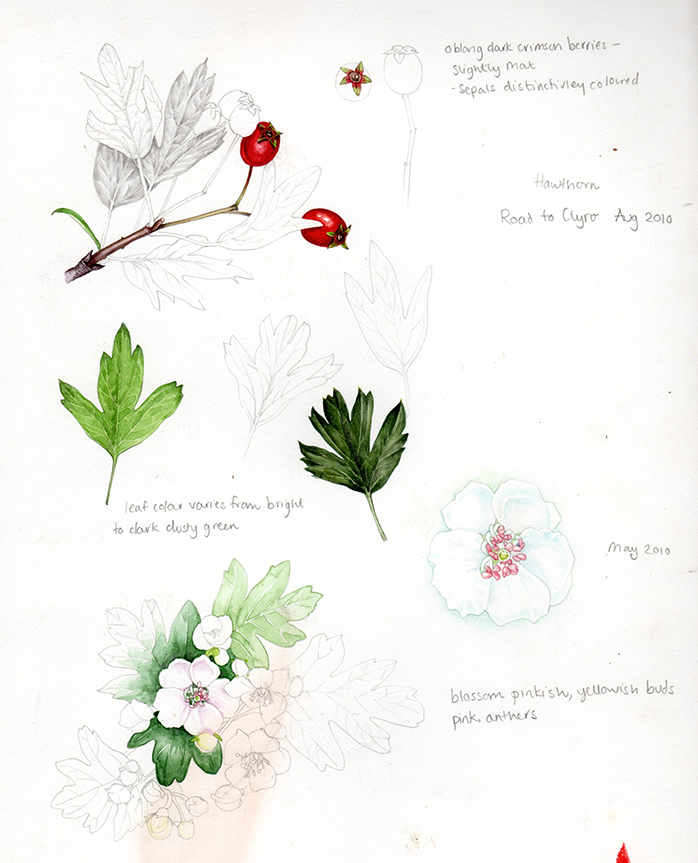The image is a vertically aligned, rectangular piece of drawing paper with a variety of detailed sketches and handwritten notes, reminiscent of a botanical study. 

In the upper left corner, there are two sketched leaves on a branch; one is shaded darker than the other. Attached to the branch are two small, round, red berries with star-shaped sepals at their ends. Below these leaves, more leaves are floating independently, with two colored in shades of green—one light and one dark—and others just outlined. An annotation next to this section reads: "A leaf color varies from bright to dark bushy green, dusty green."

Beneath this area, on the lower left side, an arrangement of flowers and leaves is depicted. Some elements are simply sketched in pencil, while others are shaded in green or pink. The central flower has very light pink petals.

In the upper right corner, more handwriting identifies the berries on the branch as "oblong, dark crimson berries, slightly matte sepals, distinctively colored". Below this, it notes "Hawthorne Road to Clyro, August 2010." Moving down the right side, there's a white flower with pink seeds nestled in the center, labeled "May 2010." Lastly, in the lower right corner, another annotation reads, "Blossom pinkish yellowish buds, pink anthers."